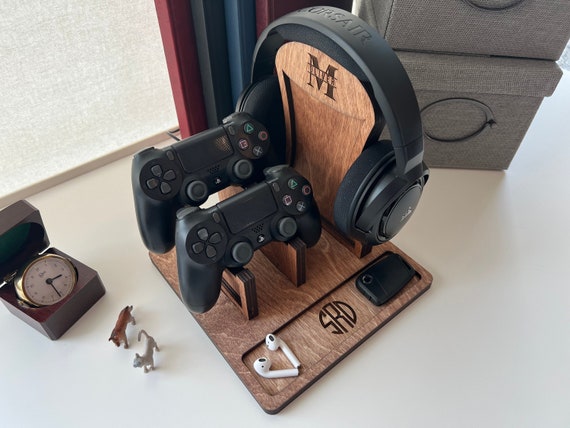The photograph showcases a meticulously arranged wooden stand, bearing the engraved initials "SRD" and "M. Oliver," designed to hold two PlayStation 4 controllers and a wireless headset. Positioned on a white desk, the wooden stand also has a pair of AirPods at its base and a car key situated to the right. To the left of the stand, there is a small golden clock encased in an open maroon box, alongside two small porcelain figurines of a cat and a dog. Adjacent to these, a pair of gray fabric storage boxes are visible. Above the stand and slightly out of focus, a decorative piece in red, gray, and blue hues adds a subtle touch. The background of the image features a white gradient, enhancing the display's aesthetics.